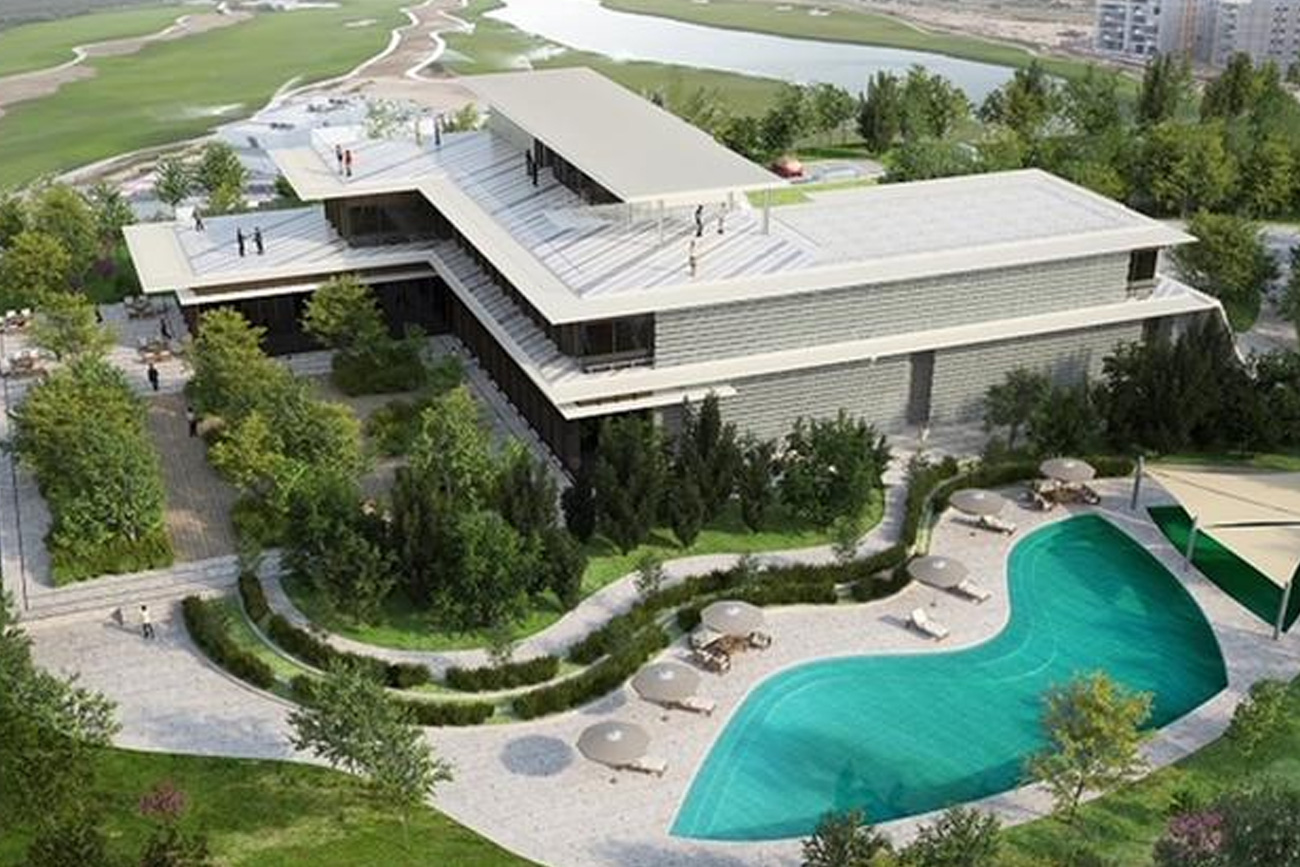The image is an aerial daytime photograph of a large property featuring a modern, geometric-shaped mansion, predominantly in a Z or L shape with an additional line extending downwards. The mansion, which resembles a sophisticated structure with a sleek white flat roof, spans three stories. The bottom story, the largest, exhibits a gray brick siding on the right and black glass windows to the left. The second level features an expansive walkable area encompassing the roof, the third level being a smaller rectangular section, possibly a bar area, notable for lacking protective borders. 

In the lower-right quadrant of the image, there is a uniquely shaped swimming pool with a wave-like contour along the top edge. The pool water exhibits a teal to bluish tone, surrounded by a light gray deck populated with sun umbrellas and lounge chairs. This deck extends towards the upper left, leading to a courtyard area in front of the mansion. 

The surrounding landscape is lush with verdant grass and numerous green trees framing the property. In the upper right background, a river is visible, adding to the picturesque setting. The photograph suggests a bustling scene with numerous people dispersed around the property, both on the ground and visible on the mansion's roof areas, indicating a possible gathering or party.